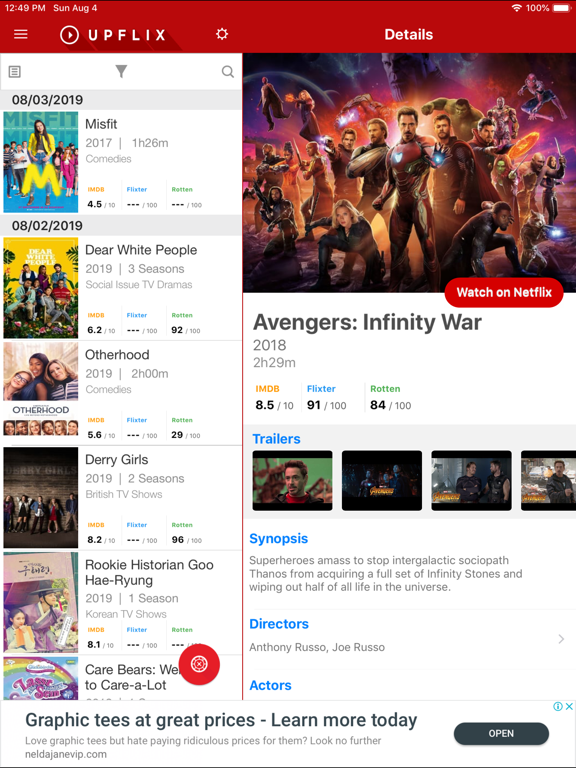The image depicts a UI design for an app or service named "UpFlix," which appears to be heavily inspired by the Netflix interface based on the use of the iconic red branding. On the left-hand sidebar, a list of movie titles is displayed, dated 8-2-2019, including "Misfit," "Dear White People," "Udderhood," "Dandy Girls," "Birkin Historian," "Hugh Raghoun," and "Care Bears: We Care A Lot." None of these movies are currently selected.

The right-hand side of the screen features a detailed pane for the movie "Avengers: Infinity War" (2018). This section provides essential information about the film: runtime (2 hours 29 minutes), IMDb rating (8.5), Clickster score (91 out of 100), and Rotten Tomatoes rating (84 out of 100). Below this information, there is a Google AdWords ad titled "Graphic Keys at Great Prices," promoting affordable graphic keys at NeldaJaneVIP.com.

An "open" button is situated on the right side of this ad. Additionally, a prominent red button labeled "Watch on Netflix" is displayed, likely serving as a main call-to-action. Beneath this button, there are headers for trailers, synopsis, and details about the directors and actors, offering further information about the movie.